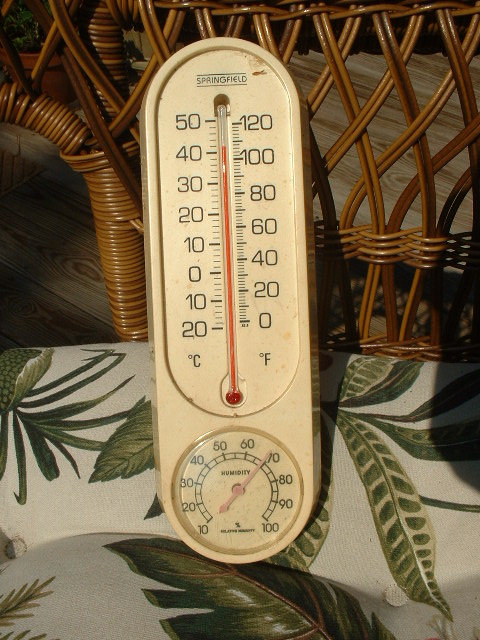The image showcases a detailed thermometer encased in an elongated, oval-shaped, pill capsule-like body. The thermometer itself is prominently displayed within this casing, with a bold red indicator showing the temperature at approximately 42 degrees Celsius. The left-hand side of the thermometer features a Celsius scale ranging from -20 to 50 degrees in 10-degree increments. Correspondingly, the right-hand side displays a Fahrenheit scale ranging from 0 to 120 degrees, indicating roughly 108 degrees Fahrenheit.

At the top of the thermometer, the brand "Springfield" is visibly marked. Below the temperature gauge, there is a humidity gauge with a measurement needle pointing to the 70% mark, signifying the current humidity level. This gauge ranges from 10 to 100.

The thermometer is placed on the seat of a wicker chair with white padding adorned with a vibrant green palm leaf pattern. The chair's woven wicker backrest creates an intricate backdrop. The scene appears to be set on a neatly laid wooden deck, adding to the rustic charm. Additionally, a potted plant is visible in the top left corner of the image, enhancing the overall natural and serene ambiance.